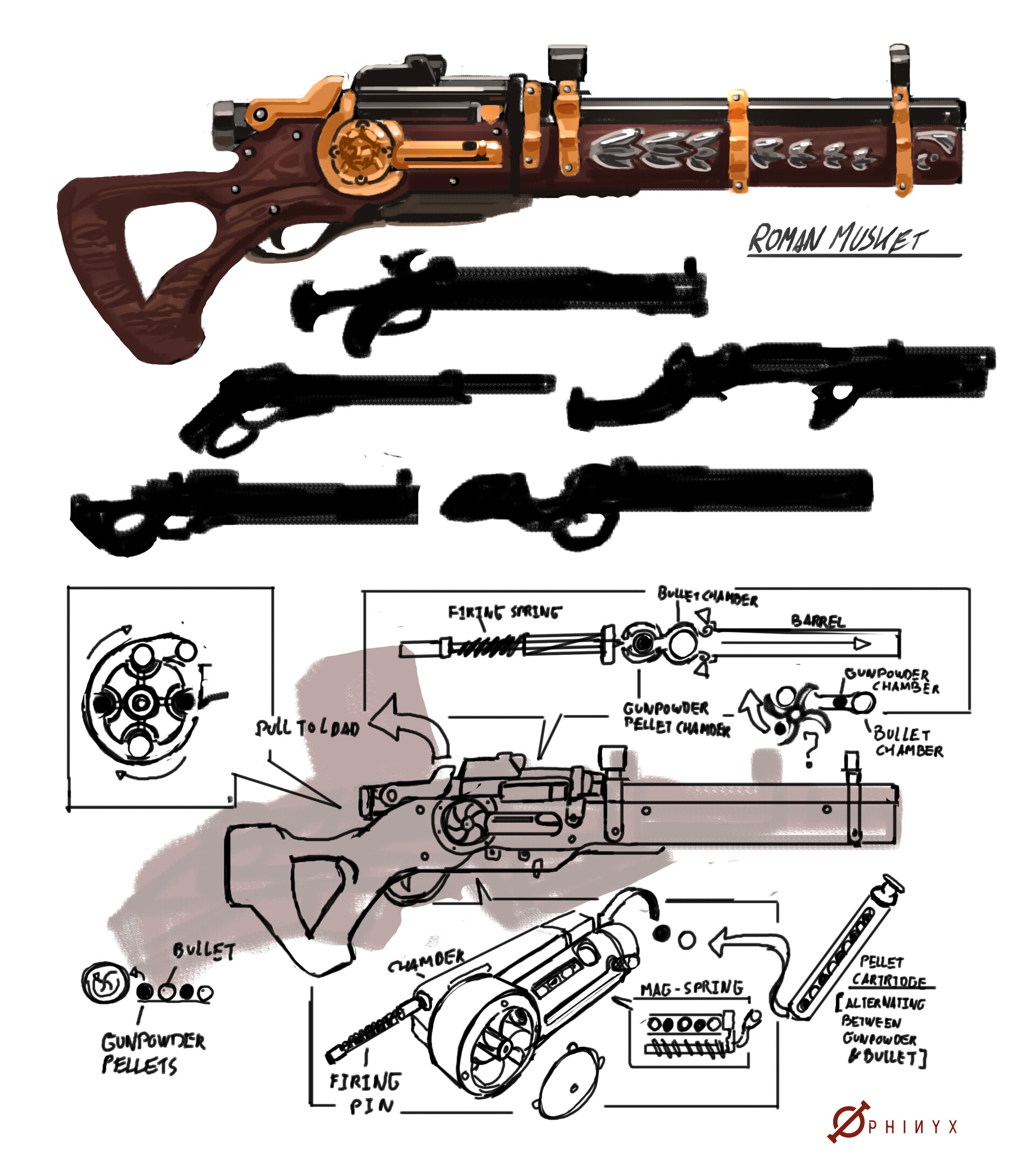The image prominently features a detailed diagram of a Roman musket at the top. This musket, rendered in a quasi-cartoonish style with markers, is primarily brown with gold-colored metal accents that clip around the barrel. The musket is labeled "Roman musket," with the text prominently underlined. Below this central figure are five black silhouettes of different types of guns, all similar in size but distinct in shape. Beneath these silhouettes is a black-and-white hand-sketched diagram illustrating the parts of the musket, including labels for the gunpowder, pellets, bullets, chamber, firing pin, and magazine spring. Additionally, the bottom right corner features a text in red with a logo displaying "Phoenix" in reverse, alongside descriptions such as "pellet cartridge," which alternates between gunpowder and bullets, and a "firing pin" callout.